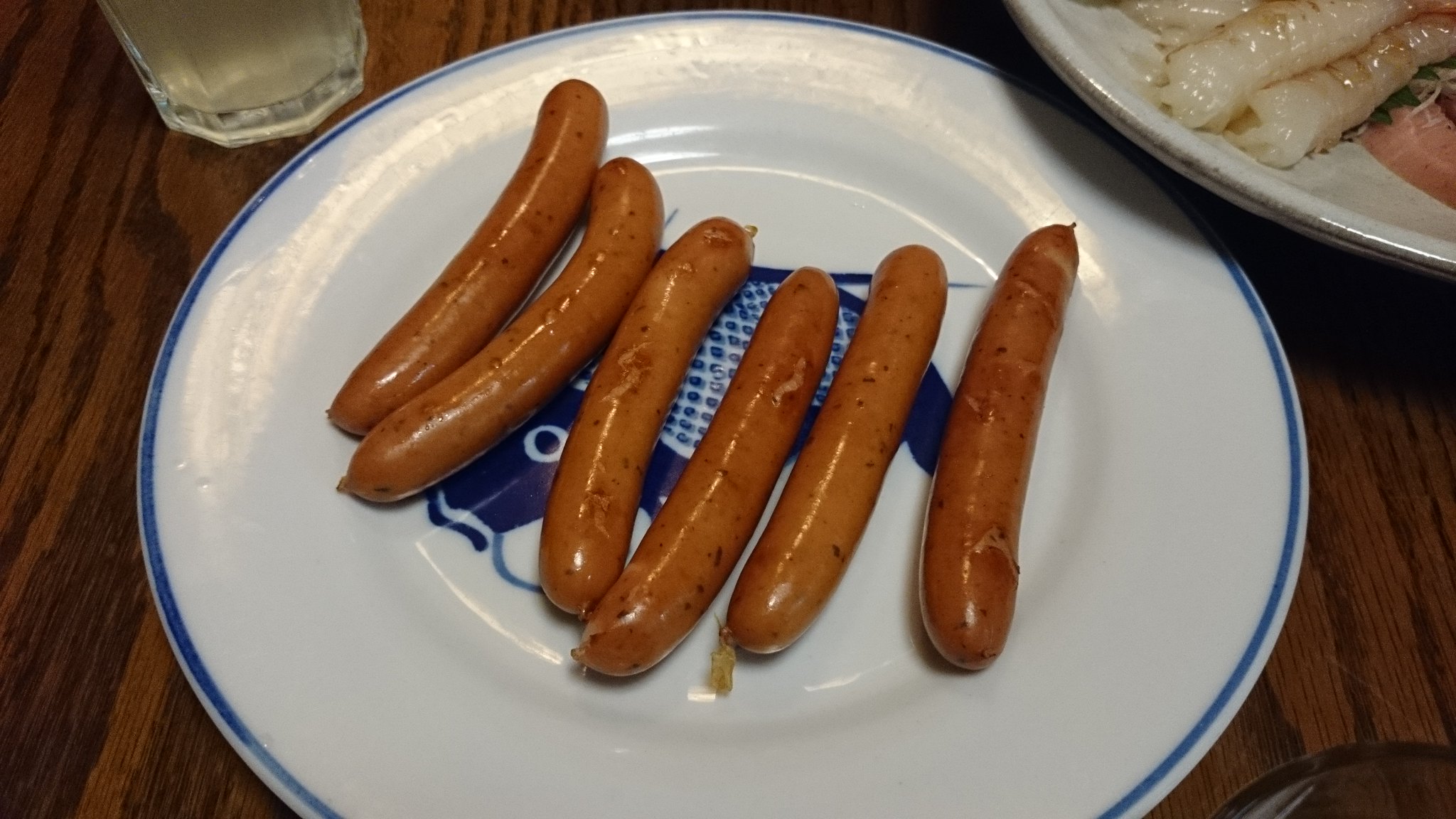The photograph features a dinner setting on a brown woodgrain table. Centered in the image is a white, round porcelain plate adorned with a blue outline around its border and a blue fish design in its center. Resting on this plate are six brown, speckled sausages, likely turkey sausages, styled vertically across the middle of the plate. The sausages appear glossy and may have been recently cooked or taken out of the package. In the upper left corner of the image, there is a glass filled with a clear liquid. To the upper right corner, there is another ceramic plate, which contains what looks like raw shrimp. The scene captures a simple yet detailed moment of food preparation or a dining setup.